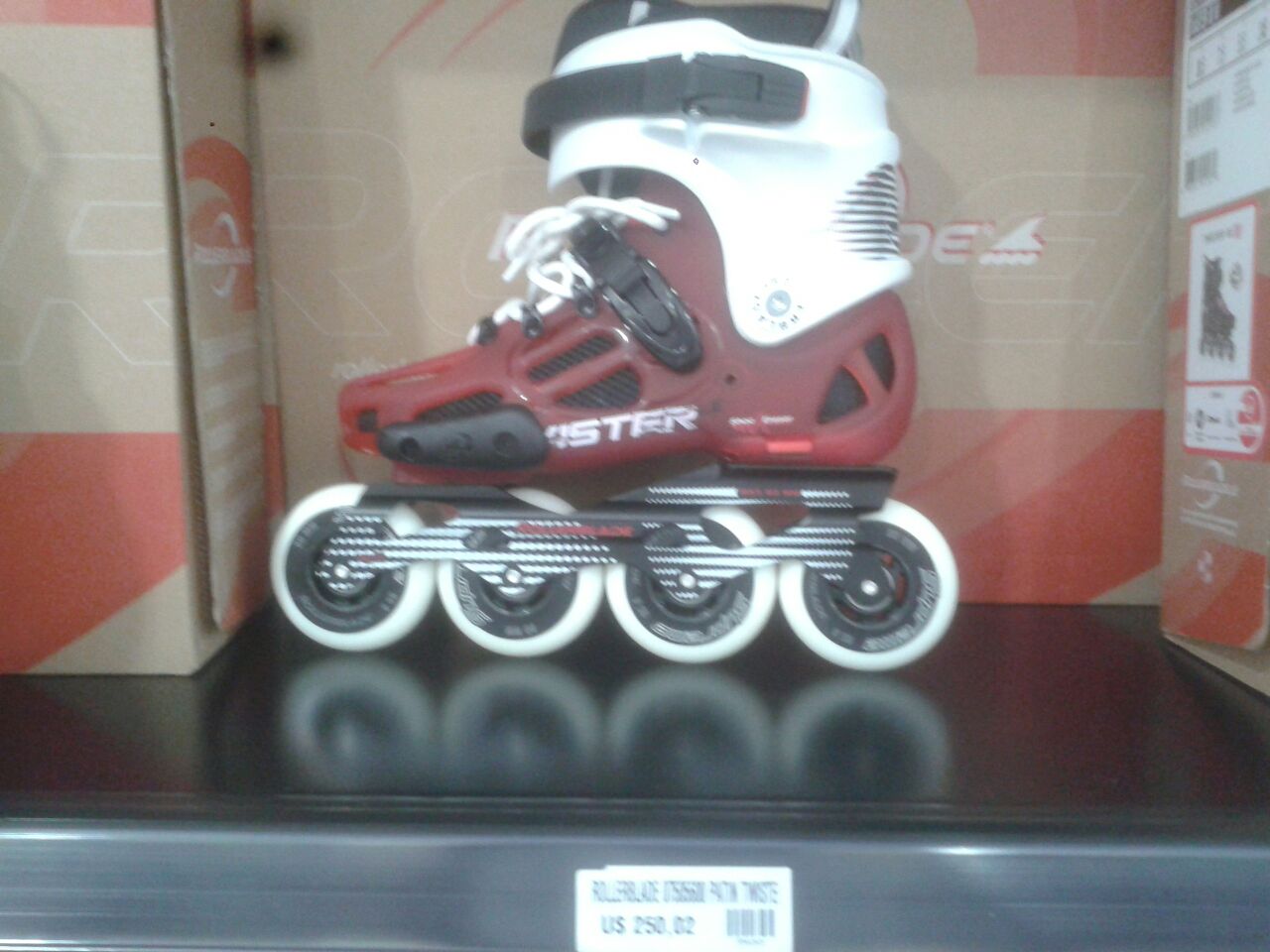This is a color photograph of an inline skate on display in a store, showcased on a shiny black wooden shelf. The skate, primarily maroon in color, features white laces and a white ankle top contrasted by black straps and a black buckle at the very top. The inline skate has four white-rimmed, dark gray wheels. The skate is surrounded by cardboard box packaging, likely containing similar skates, with some displaying orange striping. On the front edge of the shelf, there is a clearly visible white price tag with the barcode. The tag indicates "US$250.00." The skate's boot also exhibits a partially readable logo, including the letters "S-T-E-R." Reflective details of the skate's wheels can be seen on the glossy shelf surface, reinforcing the store display setting.